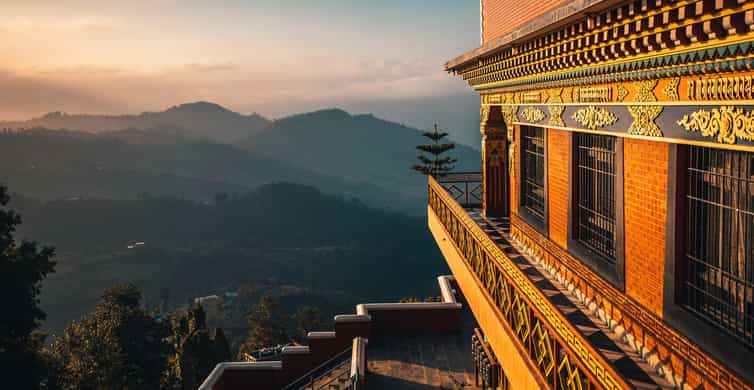The image is a wide-angle color photograph depicting a detailed landscape with a prominent ornate building that exudes an Asian, possibly Chinese or Tibetan, architectural style. Located in the highlands, the scene is dominated by rolling wooded mountains stretching into the distance under a soft gray sky, suggesting either sunrise or sunset. The building, situated on the right-hand side of the image, resembles a monastery or an imperial palace, featuring a multi-layered structure with intricate brickwork wrapped in golden-orange hues and adorned with ornate dragons and other decorations in relief beneath the roof. The facade includes black windows, some appearing barred, and a deep balcony decorated with sideways diamond trim. Steep steps or possibly the edge of a roof leads up to the building, further enhanced by a wraparound porch with similar tile work. The overall atmosphere and the architectural elements strongly convey a rich cultural heritage set against a serene, mountainous backdrop.